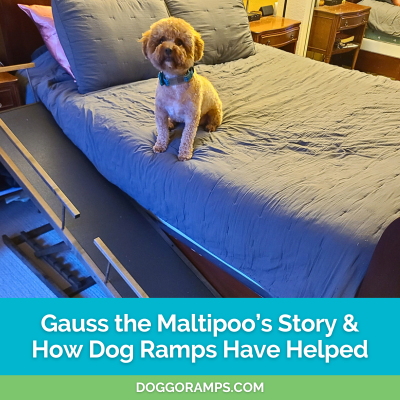The image depicts a cozy bedroom dominated by a central bed with a brown frame. The bed is neatly made with a gray blanket and matching gray pillows, accentuated by a singular pink pillow tucked behind. Perched on the bed, facing the camera, is a small and adorable brown dog, proudly sporting a green or blue collar. To the right of the bed, a ramp is visible, emphasizing its function in aiding the dog. In the backdrop, a nightstand can be seen to the upper right, contributing to the room's homely ambiance. The floor is partly visible to the lower left of the frame. Overlaying the scene is text that reads, "Gus the Maltipoo's story and how dog ramps have helped," followed by the website "DogGoRamps.com" in a green band with white lettering, making it clear that this is an advertisement for dog ramps designed to assist small dogs like Gus.